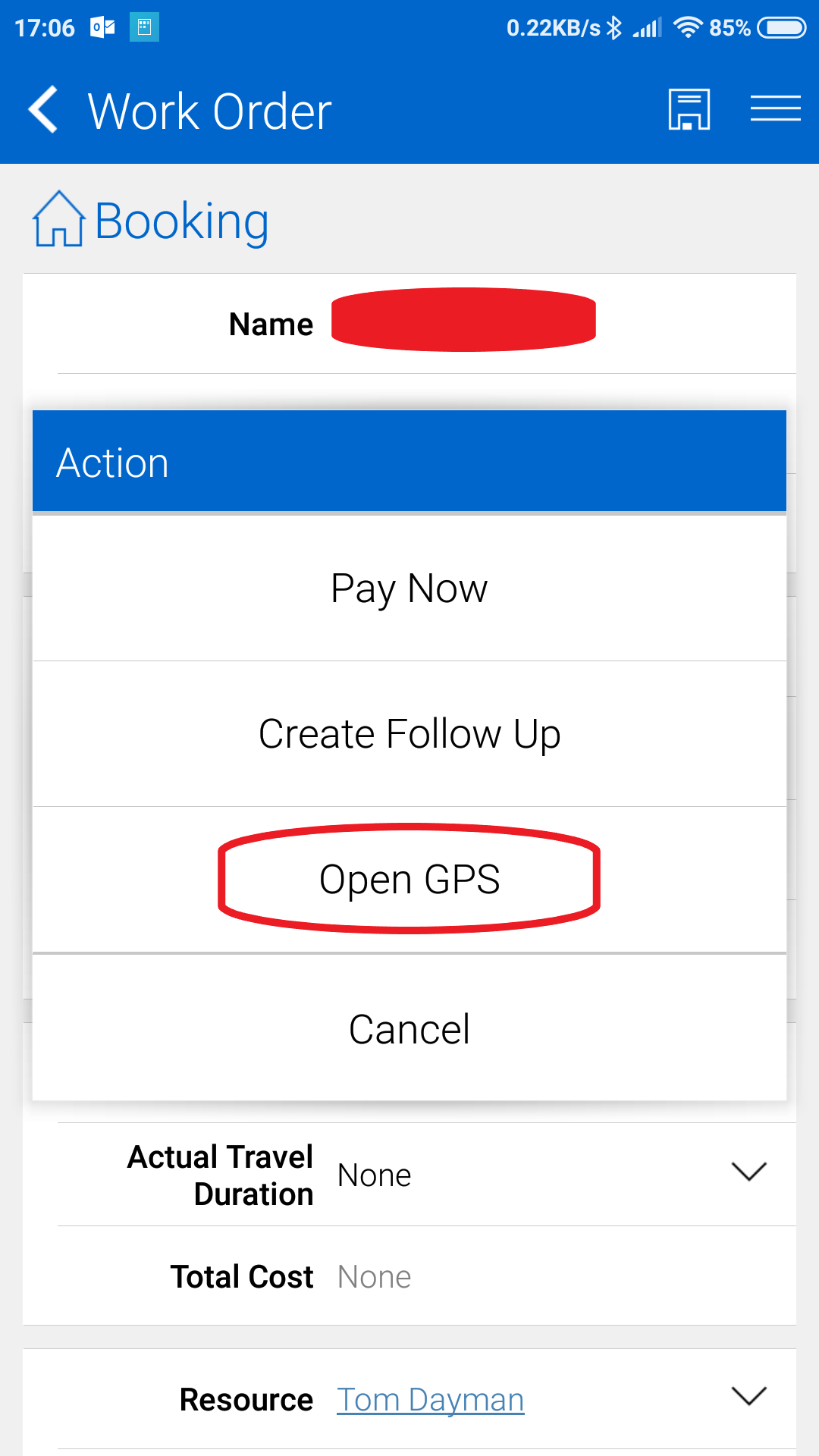A screenshot from a mobile app displays a blue header, which tints both the header and the taskbar at the top of the screen. The taskbar shows the time as 7:06, along with several icons: an Outlook icon, an unidentified teal blue square icon, a battery indicator at 85%, a full-strength Wi-Fi signal, and a one-bar cellular signal out of five. Additionally, the Bluetooth icon is active, and a data rate of 0.22 kilobytes per second is being transferred.

In the header, a left-facing arrowhead precedes the text "Work Order," accompanied by a simple line drawing of a warehouse icon and a hamburger menu represented by three horizontal lines. Below, the section labeled "Booking" is adjacent to an outlined house icon colored in blue.

On the main white field, the text "Name" appears in black font, with the actual name censored by a red mark. In another blue header are the options: "Action," "Pay Now," "Create Follow-Up," and "Open GPS" (the latter is highlighted in red). The section continues with the options "Cancel," "Actual Travel Duration: None," and "Total Cost: None." The resource is listed as "Tom Damon," which is light blue and underlined, suggesting it is a hyperlink. Two drop-down menus are present, one for "Actual Travel Duration" and another associated with the resource "Tom Damon," each indicated by a downward-facing arrow.